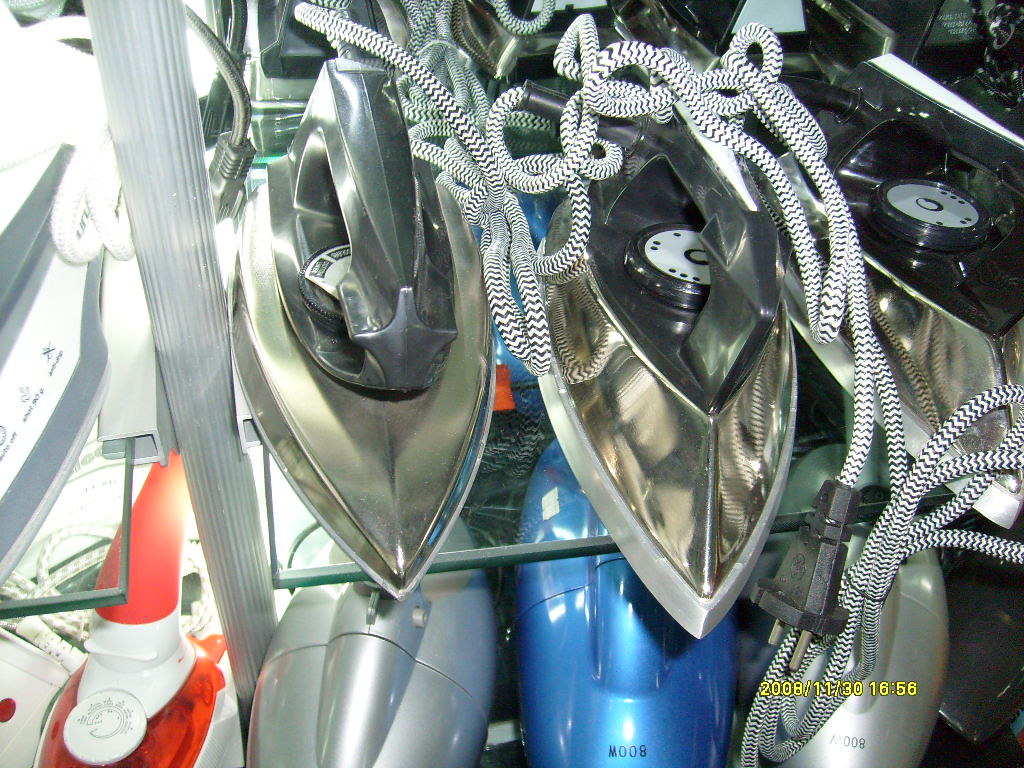This image is a detailed, close-up color photograph taken indoors with artificial lighting and a yellow timestamp in the bottom right corner reading "2008-11-30 16:58". The photograph features two shelves containing a display of vintage appliances. 

On the top shelf, a collection of old-fashioned clothing irons is showcased. These irons have a pointy shape with a stainless steel silver body, a metal surface on top, and a black portion with a dial. They feature distinctive cloth-covered cords with a black and white chevron pattern and cylindrical two-prong plugs. These irons appear identical in style and are positioned neatly on a glass shelf.

Below, a variety of small vacuum cleaners or dustbusters are seen. These appliances come in colors like red, silver, blue, and gray, with each displaying the model number "M-008". Additionally, there is an appliance with a red handle and a red top, accompanied by a white dial, possibly an alternative type of iron or steamer.

Overall, the image suggests a display case setting with lighting that highlights both the upper and lower shelves, emphasizing the vintage aesthetic of the irons and the mixed array of cleaning appliances underneath.